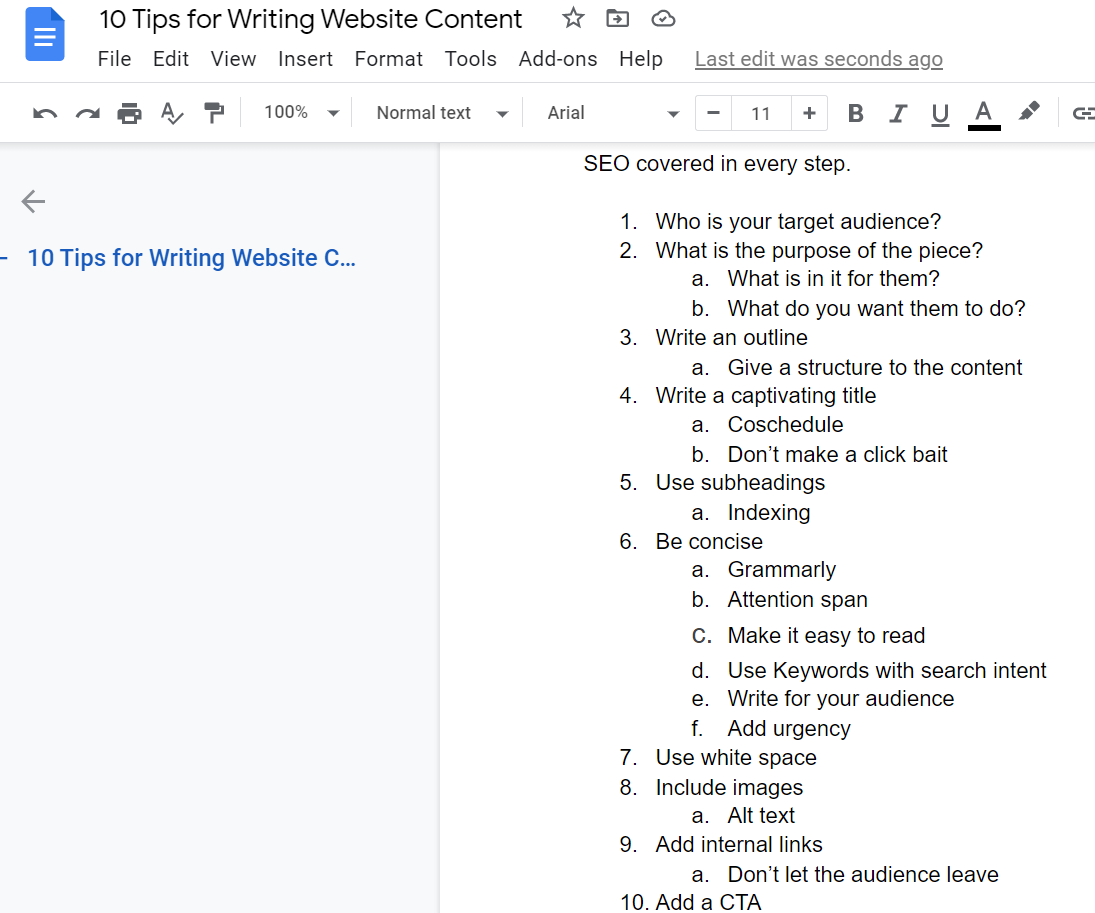The image showcases a Microsoft Word document centered on tips for writing website content. In the upper left-hand corner, a blue page icon with three horizontal lines is labeled "10 Tips for Writing Website Content." Adjacent to it are icons for star, folder, and a cloud with a checkbox. 

The top bar features standard menu headers: File, Edit, View, Insert, Format, Tools, Add-ons, and Help. To the right, it notes "Last edited was seconds ago." Directly below, an array of Word function icons is visible, including Back, Forward, Print, Text, and Paint tools. Further options include a 100% zoom drop-down menu, Normal Text drop-down, and an Arial font drop-down. There are three small boxes displaying a minus sign, "11," and a plus sign for text size adjustment. Formatting options for Bold, Italics, Underline, and Font Color are accessible, alongside a highlighter tool.

The main body of the document, positioned below these toolbars, starts with a header featuring a gray arrow pointing left and blue text that begins with "10 Tips for Writing Websites," partially cut off. Below this header, an outline details ten steps focusing on writing website content effectively, emphasizing SEO integration at each step. The document is organized into two main sections providing structured guidance on website writing.